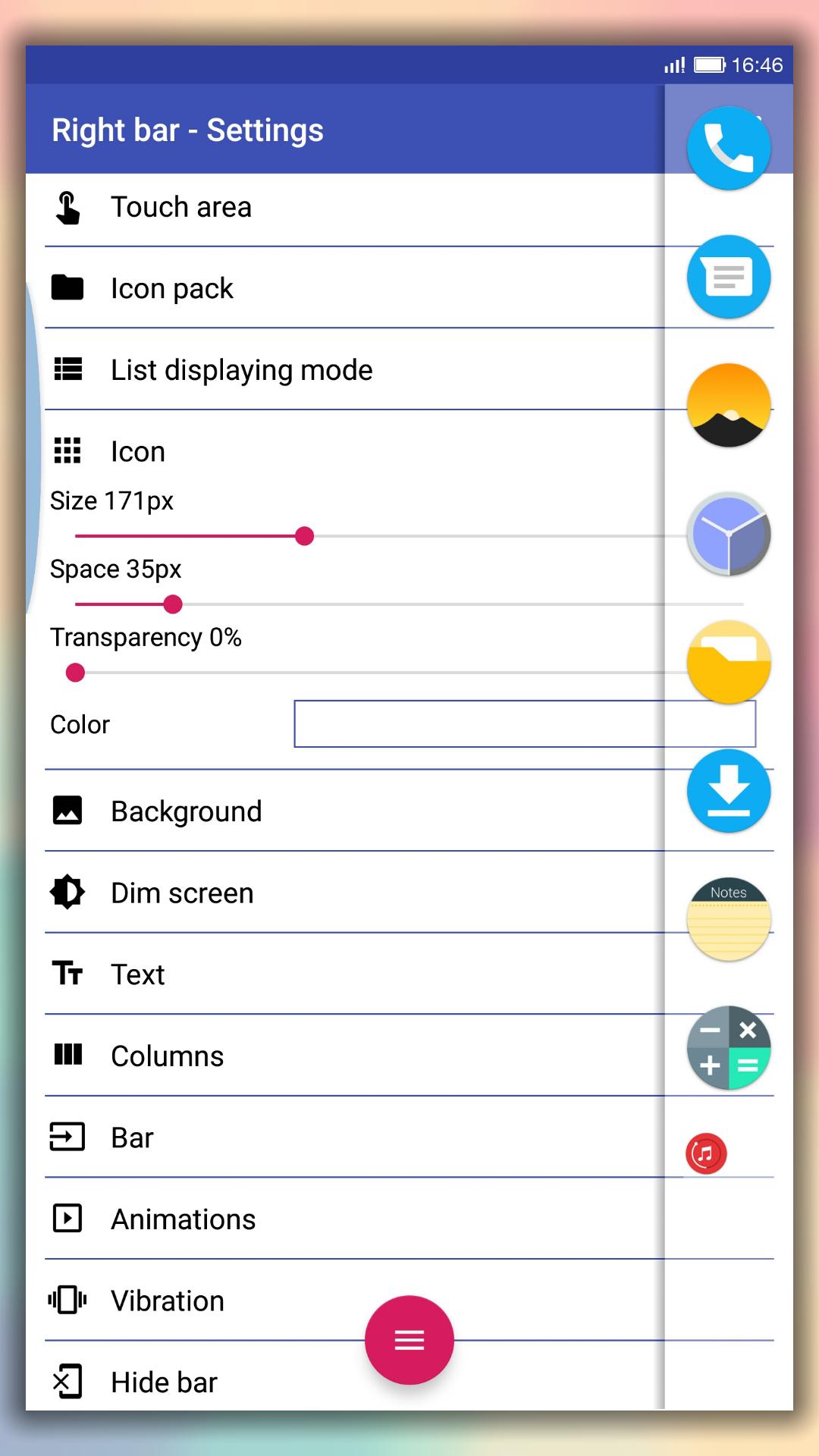In the image of the iPhone, the time displayed is 16:46 and the battery is fully charged. The iPhone's interface features a purple header at the top. Surrounding the entire phone are various vibrant colors. The screen itself exhibits a gradient of hues: transitioning from peach at the top to pink, then towards beige near the bottom, with greens running along the sides.

The interface is sectioned with white backgrounds bordered by gray lines. The sections read: "Touch Area," "Icon Pack," and "List Displaying Mode." The detailed settings include text indicating "Icon Size: 171px," "Space: 35px," and "Transparency: 0%," with corresponding pink bars and pink circle markers at the ends. There's a labeled "Color" box, which is white, followed by settings for "Background," "Dim Screen," "Text," "Columns," "Bar," "Animations," "Vibrations," and "Hide Bar." In the middle, between "Vibration" and "Hide Bar," is a pink circle icon featuring three white lines.

On the right side of the screen, a vertical array of icons is observed in varying colors: blue, gold, blue again, beige, and a multi-colored one at the bottom.